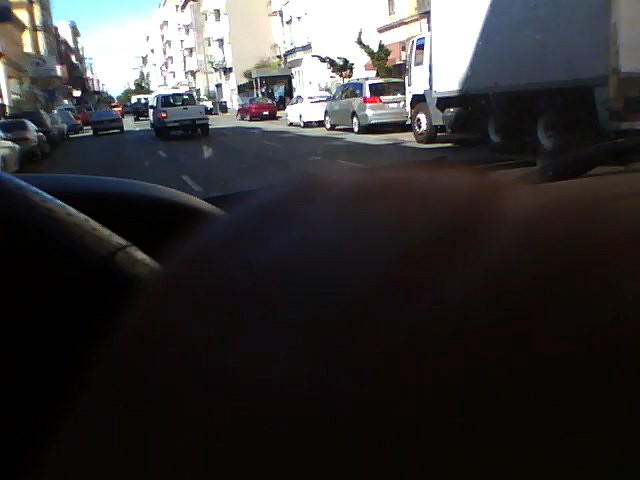Taken from inside a car, the photo captures a bustling city street from the perspective of the driver's seat. Part of the black steering wheel and the dashboard occupy the foreground, with a person's hand partially visible on the wheel. The street outside consists of three lanes, teeming with daytime traffic and lined with parked cars on either side. To the right, a red car is parked with a white car behind it, while the left side of the street shows more cars neatly lined up.

Several multi-story apartment buildings with balconies flank both sides of the road, contributing to the busy urban atmosphere. A gray minivan travels in the far-left lane, followed by a white delivery truck casting a shadow across part of the street. The middle lane features a white truck, with other vehicles ahead in steady progression. The photo captures the essence of city life, with tall buildings and an array of vehicles moving and parked along the thoroughfare.